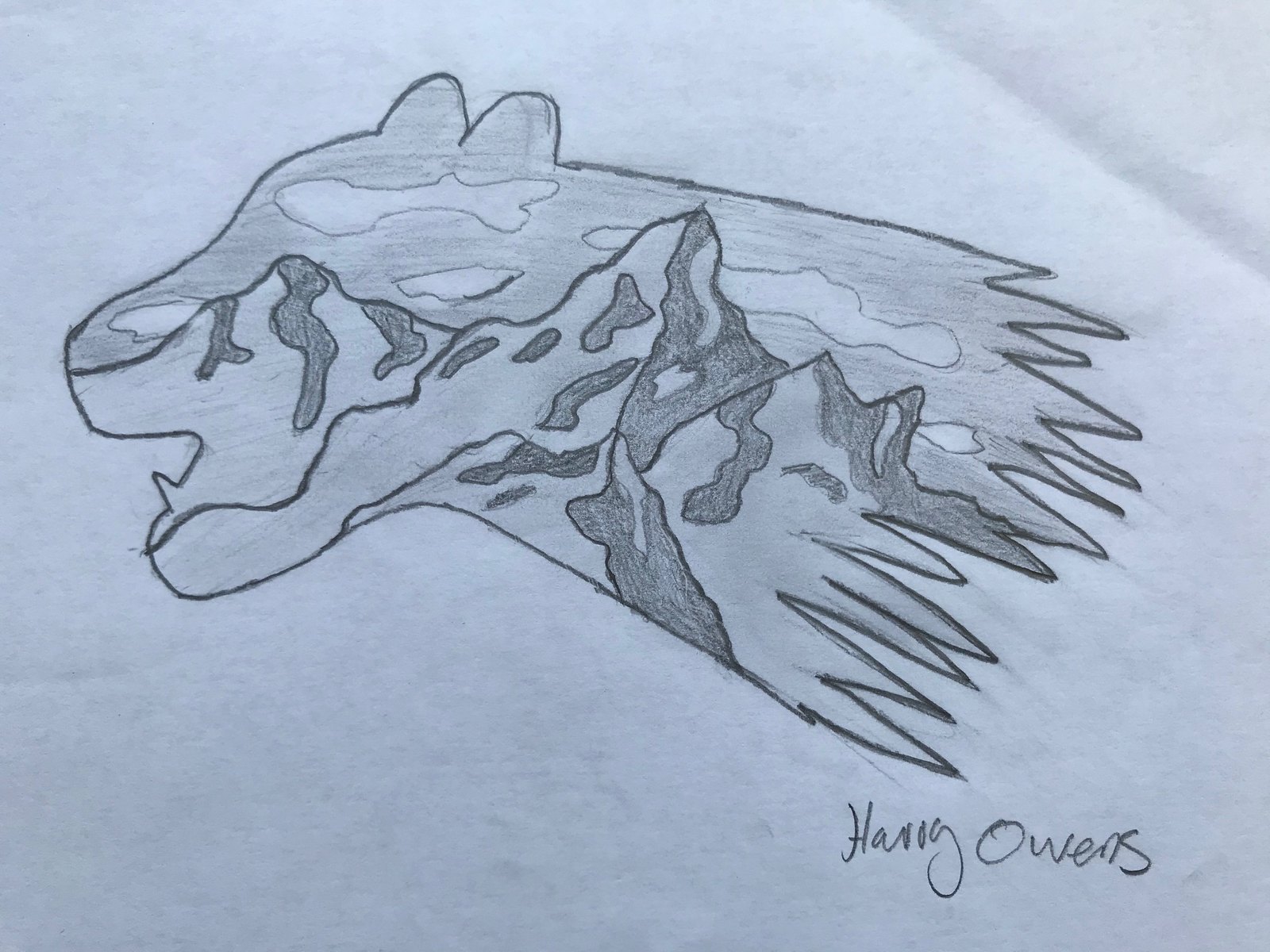This is a detailed photograph of a drawing on a white piece of paper, rendered intricately using various shades of lead pencil. The artwork depicts the head and neck of a cheetah, meticulously outlined with bold, dark, and thick lines. The interior showcases elaborate shadings, creating a sense of depth and texture. Dark, heavily outlined spots embellish the cheetah's fur, enhancing the lifelike representation of the cheetah's distinctive pattern despite the monochromatic palette. The cheetah's mouth is open, revealing a visible tooth, and its two prominent ears are distinctly detailed at the top of the head. The neck culminates in a series of sharp, spiky strokes, adding a dynamic finish to the drawing. The artist, Harry Owens, has signed their name prominently in the bottom right corner, marking their remarkable pencil work.